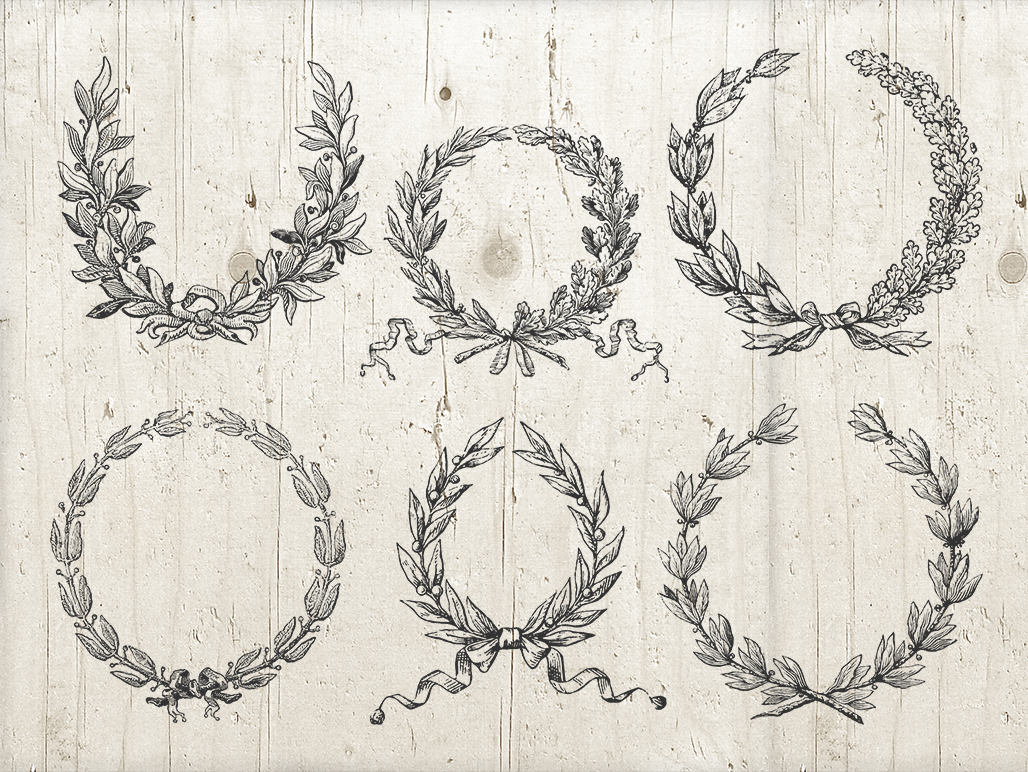This image showcases an illustration of six meticulously detailed, black-and-white wreaths set against a rustic, light beige and gray wooden background with natural knots and cracks. The wreaths, arranged with three on the top and three on the bottom, exhibit various designs and shapes, each accompanied by festive ribbons that add a touch of flair. 

1. The upper left wreath is a horseshoe shape adorned with leaves and a central bow at the bottom.
2. To the right, there is a typical circular wreath with a long ribbon dangling from the bottom.
3. The third wreath on the top row features two-tone olive branches, curving upwards from left to right, and a bottom ribbon.
4. On the bottom row, the leftmost wreath is almost floral in design, with a bow at the bottom.
5. Next to it, a small wreath circle is encircled by a prominent ribbon and bow.
6. The final wreath on the far right is a full circle of olive branches with no bow, distinguished by its simple elegance.

While all wreaths feature leaves of diverse shapes, the bottom center wreath stands out as the most festive, with its particularly curly ribbons that add extra flair and a fun vibe to the illustration.